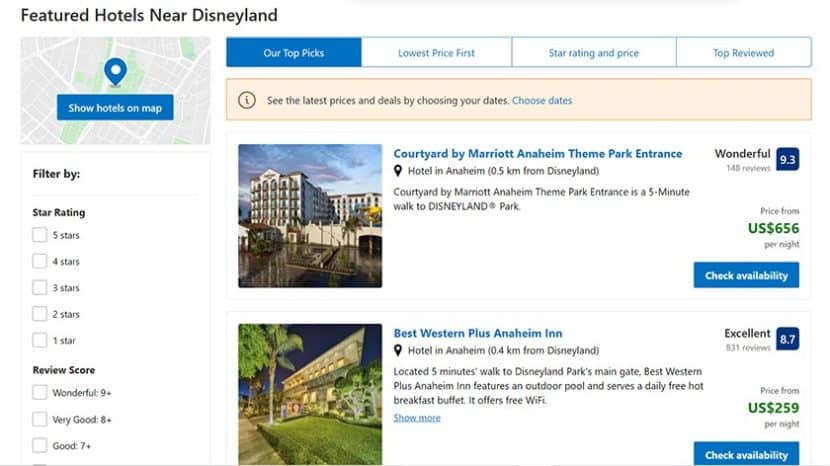"Horizontal image displaying a well-organized webpage, likely viewed on a computer or smart device, for selecting hotels near Disneyland. The webpage features a white background. At the top-left corner in bold black text, the heading reads 'Featured Hotels Near Disneyland.' Below this, a small map with a blue icon featuring a white circle in the center is labeled 'Show Hotels on Map.'

Further down, bold text 'Filter By' is visible, followed by options for filtering hotels by Star Rating, allowing selections from one to five stars. Another section labeled 'Review Stars' offers additional filtering options, including 'Wonderful (9+),' 'Very Good (8+),' and 'Good (7+),' though none are selected.

Across the top-middle portion, tabs include 'Our Top Picks' (highlighted in blue), 'Lowest Price First,' 'Star Rating and Price,' and 'Top Viewed.' Below this navigational bar, a prominent peach-colored rectangle contains black text stating, 'See the Latest Prices and Deals by Choosing Your Dates,' with an adjacent blue 'Choose Dates' button.

In the main body of the page, the Courtyard by Marriott Anaheim Theme Park Entrance is featured first, with its name in blue, proximity details to Disneyland, review score, price, and a 'Check Availability' button. Directly below this listing, a similar format presents the Best Western Plus Anaheim Inn with corresponding details and a 'Check Availability' button in blue."